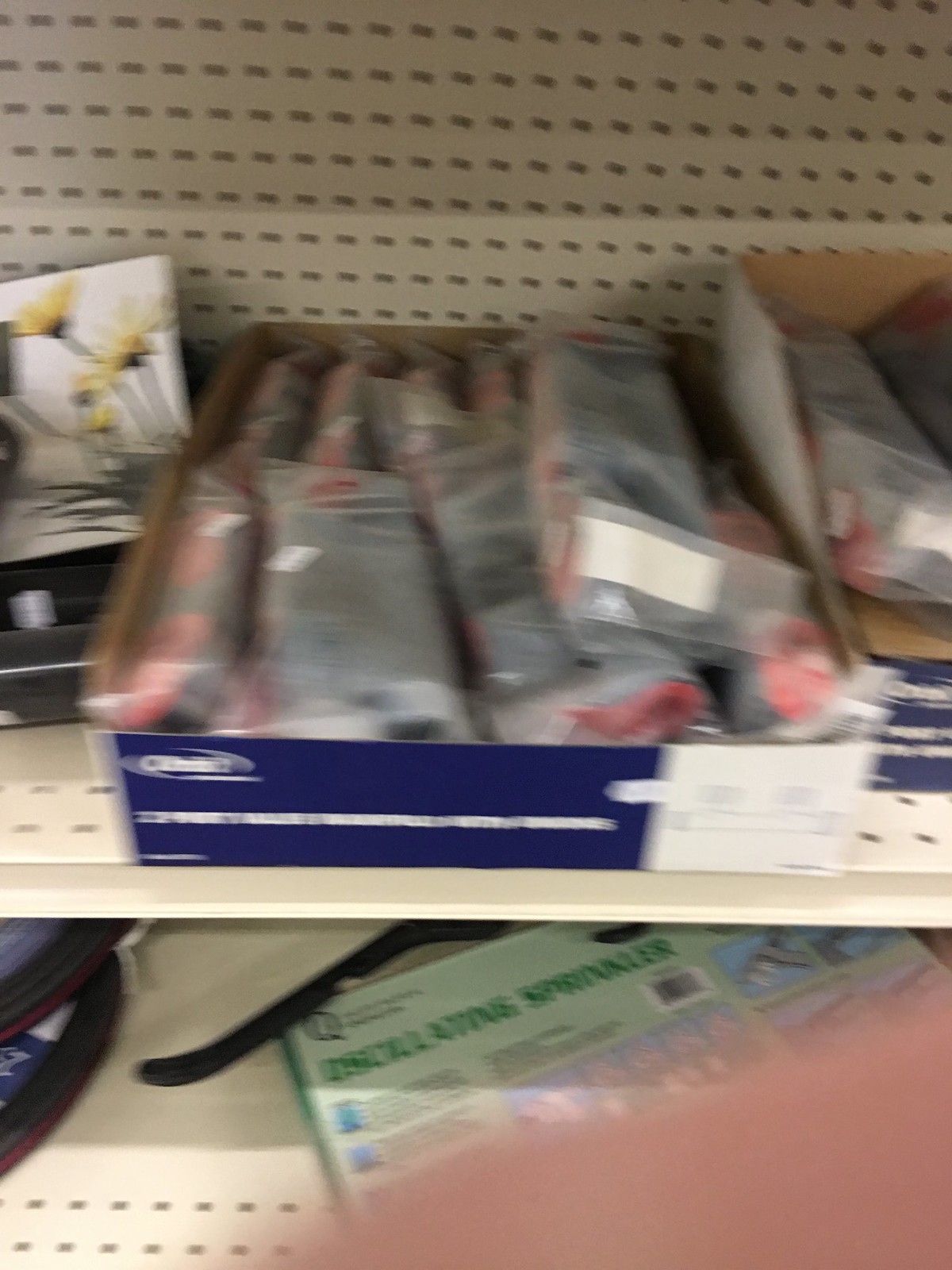This image, although slightly blurred, captures a section of retail store shelving. The shelves, painted a cream color, house a variety of products. On the top shelf, there is a cobalt blue box with white writing containing multiple smaller packages. These packages are primarily dark gray with orange trim. Next to this blue box, on the right side, are several opaque white plastic packages. To the left of the blue box, a card is placed, featuring a white background decorated with yellow daisies. The daisies have bright yellow petals and green stalks, which extend from the lower right corner towards the middle top of the image, adding a touch of natural beauty to the scene.